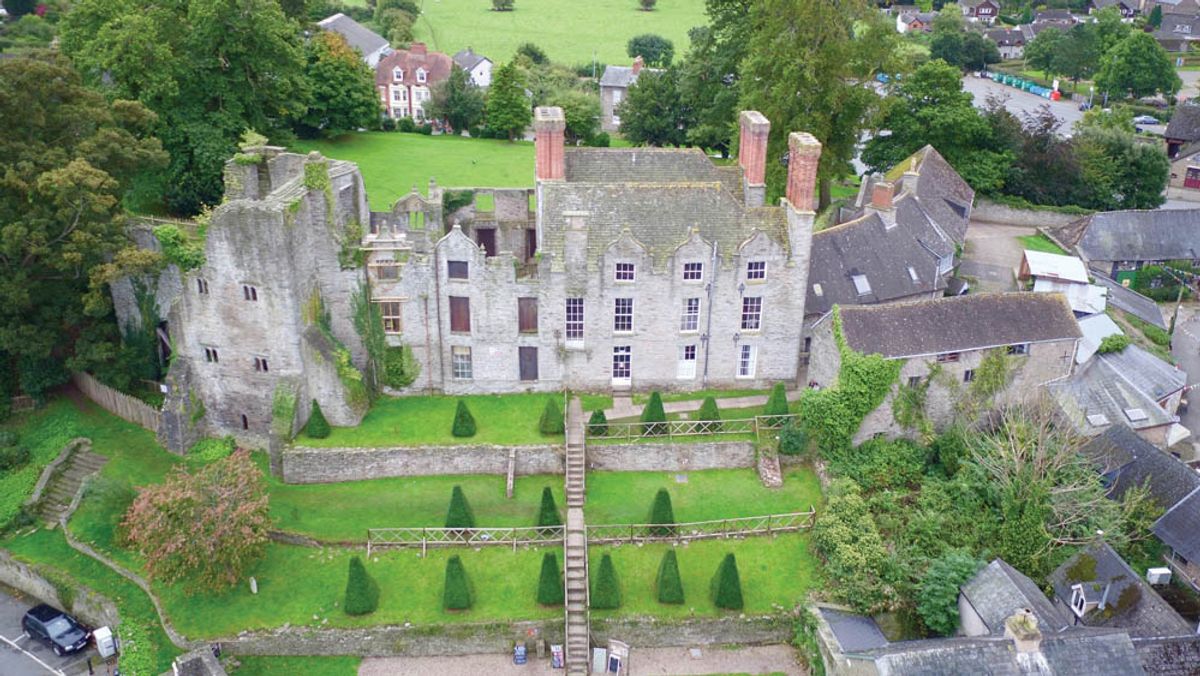This aerial photograph captures a grand, largely roofless stone manor house, possibly in England, from a height akin to that of a helicopter. The building, with a vast and lateral footprint, spans three to four stories adorned with mullioned windows. Its right side features three prominent brick chimneys, while the left side appears more deteriorated, suggesting ruin-like conditions. Notably, greenery and moss overtake sections of the structure, particularly evident on a few buttresses and along the roofless areas. Cascading plants overhang the top, complementing the lush surroundings.

The foreground reveals a meticulously maintained lawn interspersed with tiered rows of perfectly conical pine trees, accentuating the symmetrical landscaping. A gray stairwell ascends through three levels of lawn, leading up to the main entrance of the manor. Nearby, glimpses of a parking area with a black car and a white cubicle add modern touches to the otherwise historical scene.

Surrounding the manor, present-day buildings with visible rooflines and occasional chimneys form a neighborhood backdrop. The distances are filled with greenery, additional houses, and roads, blending seamlessly into the extensive lawns and trees that frame this panoramic view.